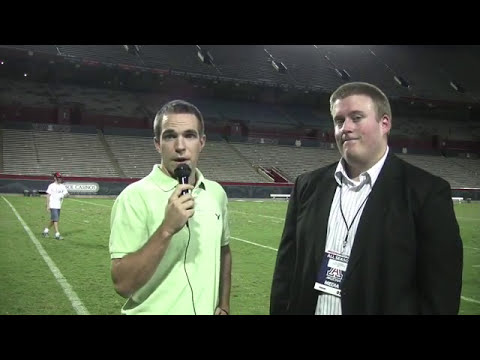In the image, two men are prominently featured standing on a football or soccer field in an empty stadium. The man on the left, who appears to be a reporter, is holding a microphone and clearly speaking while looking directly at the camera. He is dressed in a neon lime green short-sleeve polo shirt. The man on his right, who seems to be the interviewee, is wearing a black sport coat over a white collared shirt, complemented by a lanyard with an indistinguishable pass. Both men have short dark hair. The interviewee's expression is rather neutral, with a hint of annoyance. In the background, the stadium seats are completely empty, and a single person, likely a groundskeeper, can be seen walking across the field. This individual is clad in a white t-shirt, shorts, and a hat. The overall scene appears to be a screenshot from a video, distinguished by its vibrant colors—greens, whites, blacks, and a mix of peach, blue, red, and gray.